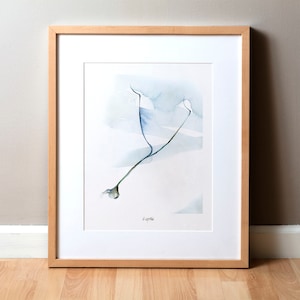This image shows a piece of framed artwork propped up against a taupe-colored wall with a white baseboard. The frame is portrait-oriented and made of light wood, matching the light-colored hardwood floor it rests on. The artwork inside the frame is bordered by a white matte. The painting itself features a white background with a watercolor composition dominated by hues of blue. Towards the top right, there is a light blue wash that transitions into darker blue lines extending downwards, forming a Y shape that tapers off toward the bottom left, resembling roots or a stethoscope. Although the exact subject of the painting is ambiguous, the minimalist and abstract nature of the watercolor piece is highlighted. There is also a signature located at the bottom of the artwork, indicating it might be an amateur creation or simply a piece open to interpretation, underscoring the idea that art is in the eye of the beholder.